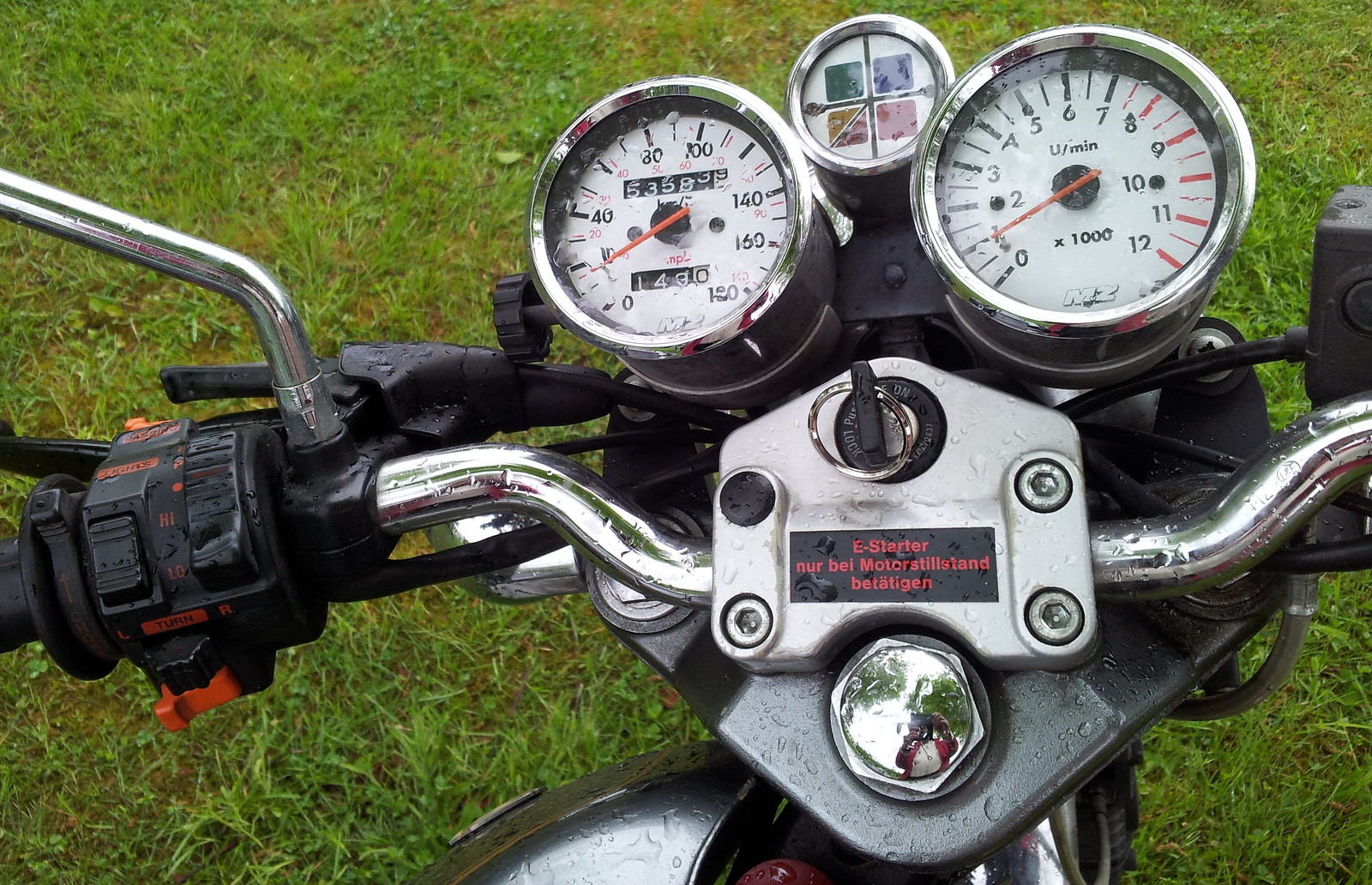The image features a close-up of motorcycle handlebars adorned with various instruments and controls. The handlebars are predominantly black with silver metal accents. Positioned prominently in the center are three gauge-like displays. The largest, a traditional speedometer, is marked with numbers ranging from 0 to 180. To its right, a secondary gauge is divided into four colored quadrants: green in the top left, blue in the top right, red in the bottom right, and yellow in the bottom left, each color segmented into smaller squares. On the far right, another dial measures from 0 to 12.

Beneath the gauges, the ignition slot features the label "E Starter" alongside text that appears to be in German. The key is inserted into the ignition. Reflecting in the bolt below the ignition is a silhouetted figure of the person taking the photo, dressed in a red jacket, with trees visible in the background.